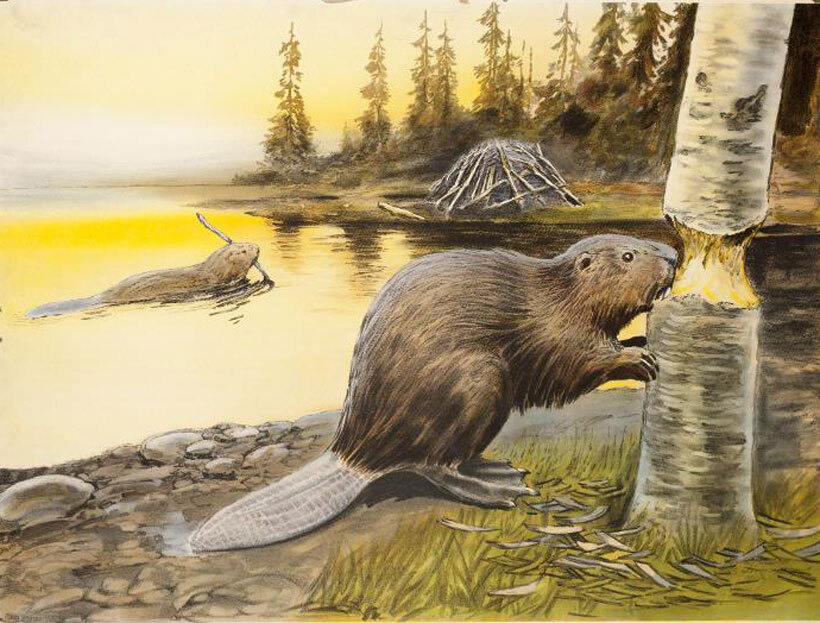In this digital painting of a nature scene, two beavers are depicted in a detailed and vibrant environment. In the foreground stands a beaver on its large, flat tail and hind legs, with its front paws resting on a tree trunk as it gnaws through the bark, creating a yellow exposed inner core in a distinctive, almost apple-core shape. The beaver's body, facing to the right, is positioned near the muddy, rock-strewn shore of a pond or lake. The light gray or white ash-like tree trunk leans toward the right, and to the right of the tree, a patch of wild grass grows. In the water to the left, another beaver swims away from the viewer, a branch clenched in its mouth, heading towards a large pile of sticks and logs that form a dam or beaver lodge on the opposite shore. The water shimmers with golden reflections from the sun, which is centrally depicted, casting its light through the trees and creating a luminous contrast between the lighter foreground and the darker background. The scene is framed by spindly evergreen trees and tall trunks, under a sky that transitions from yellow at the top to a light horizon. Dominated by hues of brown, green, yellow, and gray, the painting captures the industrious daily life of the beavers amidst the tranquil, yet dynamic, woodland backdrop.